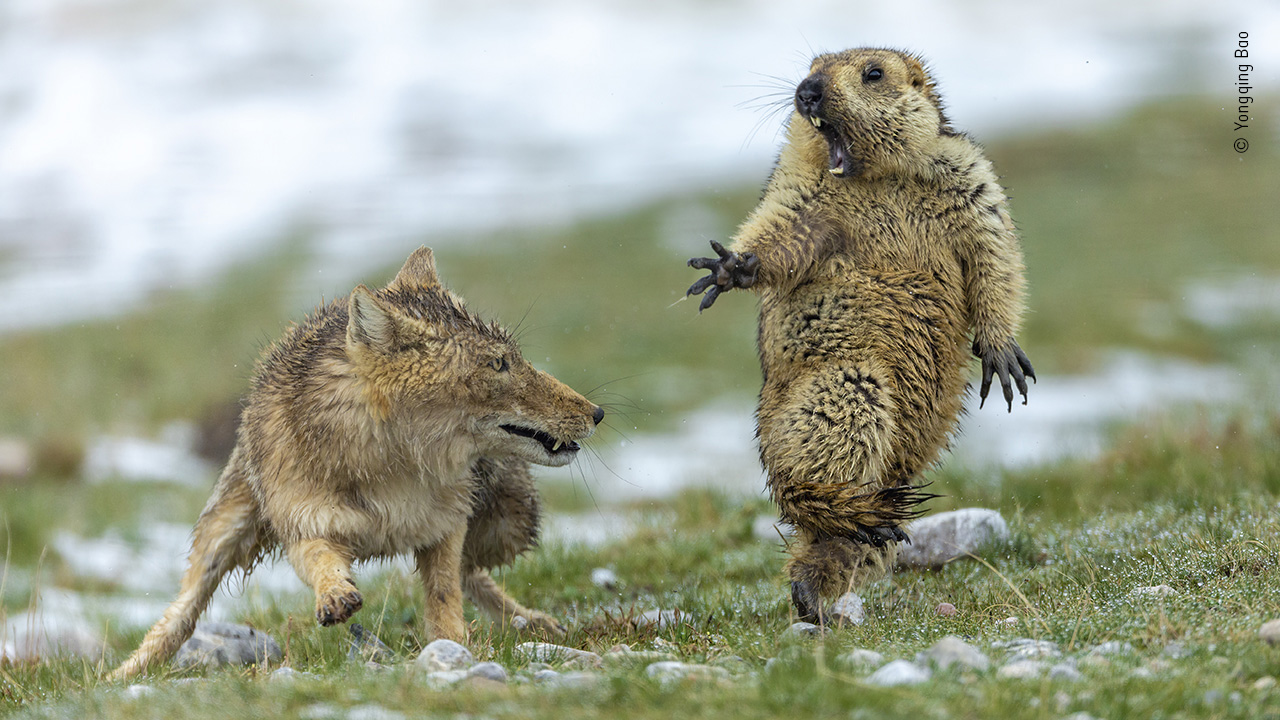In this composite photograph, we see two animals set against a grassy field—one resembling a brown wolf or fox and the other a groundhog or beaver. The wolf-like creature is positioned on our left, gazing intently at the groundhog-like animal on the right. The groundhog stands on its hind legs, appearing terrified with its mouth open and teeth visible, as if letting out a scream of fear. Despite the realistic backdrop, the photograph's composition creates an unnatural perspective; the groundhog seems disproportionately large compared to the wolf, leading one to suspect the image was digitally manipulated. The two creatures, both brown in color, are surrounded by rocks and sparse grass, possibly with some snow in the background. This intriguing, albeit unrealistic, scene captures a moment that blends elements of both predator-prey dynamics and artistic digital alteration.